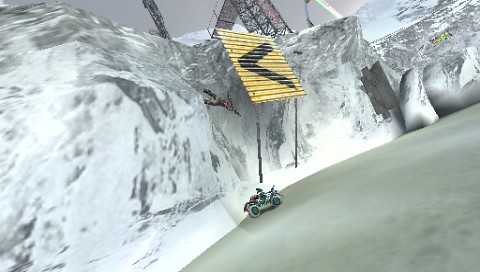In this vividly detailed screenshot from a snowmobile racing video game, a player-controlled snowmobile is depicted crashing into a wall of ice, set against a stark and wintry landscape. The icy backdrop features a prominent yellow sign with a black arrow pointing left, indicating a sharp turn that the player evidently missed. Above, the sky is dark and ominous, adding to the challenging and intense atmosphere of the game. The snowmobile's bold and swift maneuvering contrasts sharply with the cold, unforgiving environment, emphasizing the dramatic moment of impact.